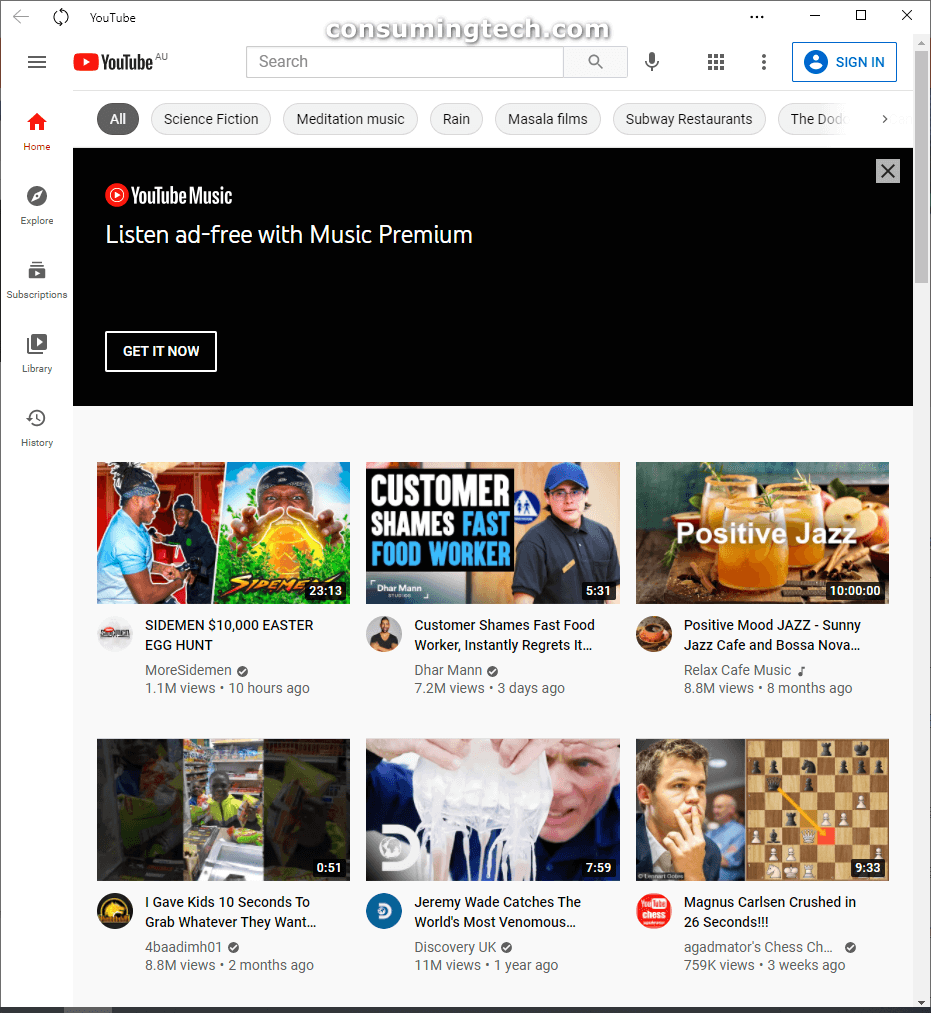The image is a vertical rectangle, displaying a browser or the YouTube app. At the top, the familiar YouTube logo, featuring a red box with a white play symbol, is prominently visible. Below the logo is a search field, allowing users to type in their queries. Above the search field, the webpage title "consumingtech.com" is displayed. To the right of the search bar, there is a microphone icon, a nine-square matrix icon, three vertically-aligned dots, and a "Sign In" button.

On the left side of the screen, there is a vertical menu with various icons: Home, Explore, Subscriptions, Library, and History, with the Home icon currently selected. 

The main content area starts with a promotional black box for YouTube Music, offering an ad-free experience with Music Premium, accompanied by the call-to-action "Get it now." Below this promotion, there are six video thumbnails. The videos include titles such as "Easter Egg Hunt," "Customer Shames Fast Food Worker, Instantly Regrets It," "Positive Mood Jazz," and "Sunny Jazz Cafe," among others.